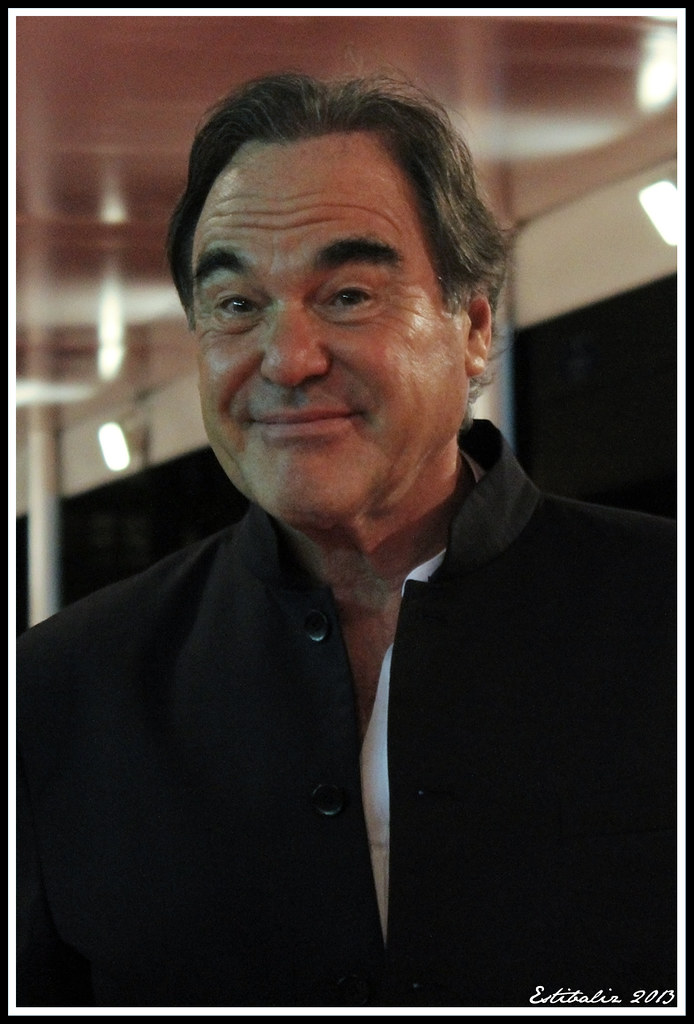The image captures an older gentleman with a warm, satisfied smile and an oval-shaped face, characterized by puffy, prominent cheeks and dark, slightly combed back, salt-and-pepper hair that does not quite reach his ears. His clean-shaven face shows deep smile lines, suggesting he's often in good spirits. He has dark eyes and eyebrows. He is dressed in a black jacket, resembling a chef's coat with a short collar and large buttons, the top three of which are undone, revealing a white shirt underneath. The background is blurry but appears to be an indoor setting, possibly a large room or restaurant, with some indistinct columns and lights. In the bottom right corner of the image, a cursive signature and the year "2013" can be seen, though the text is difficult to decipher, possibly reading "Estibaliz." The focus of the photo is clearly on the man, giving an impression of candid spontaneity.